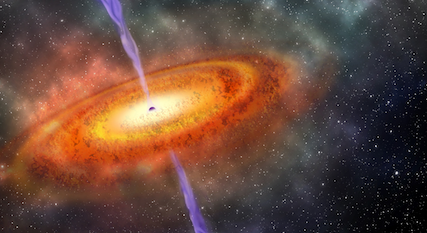This captivating color image from outer space, with uncertain origins—possibly from a real-life capture or a movie or TV show—features a mesmerizing glowing orange and yellow spiral slightly left of center. At the heart of the spiral is a bright, vibrant yellow core. Emanating from both the top and bottom of this core is a wavy purple line, adding a dynamic element to the scene. Surrounding the spiral are ethereal, cloudy masses that enhance the sense of depth and space. The backdrop is a deep, inky black sky, richly adorned with numerous twinkling stars. The photograph has a widescreen aspect ratio, emphasizing the expansive cosmic landscape. Notably, the image contains no people, animals, writing, or vegetation, allowing the viewer to focus entirely on the stunning astronomical spectacle.